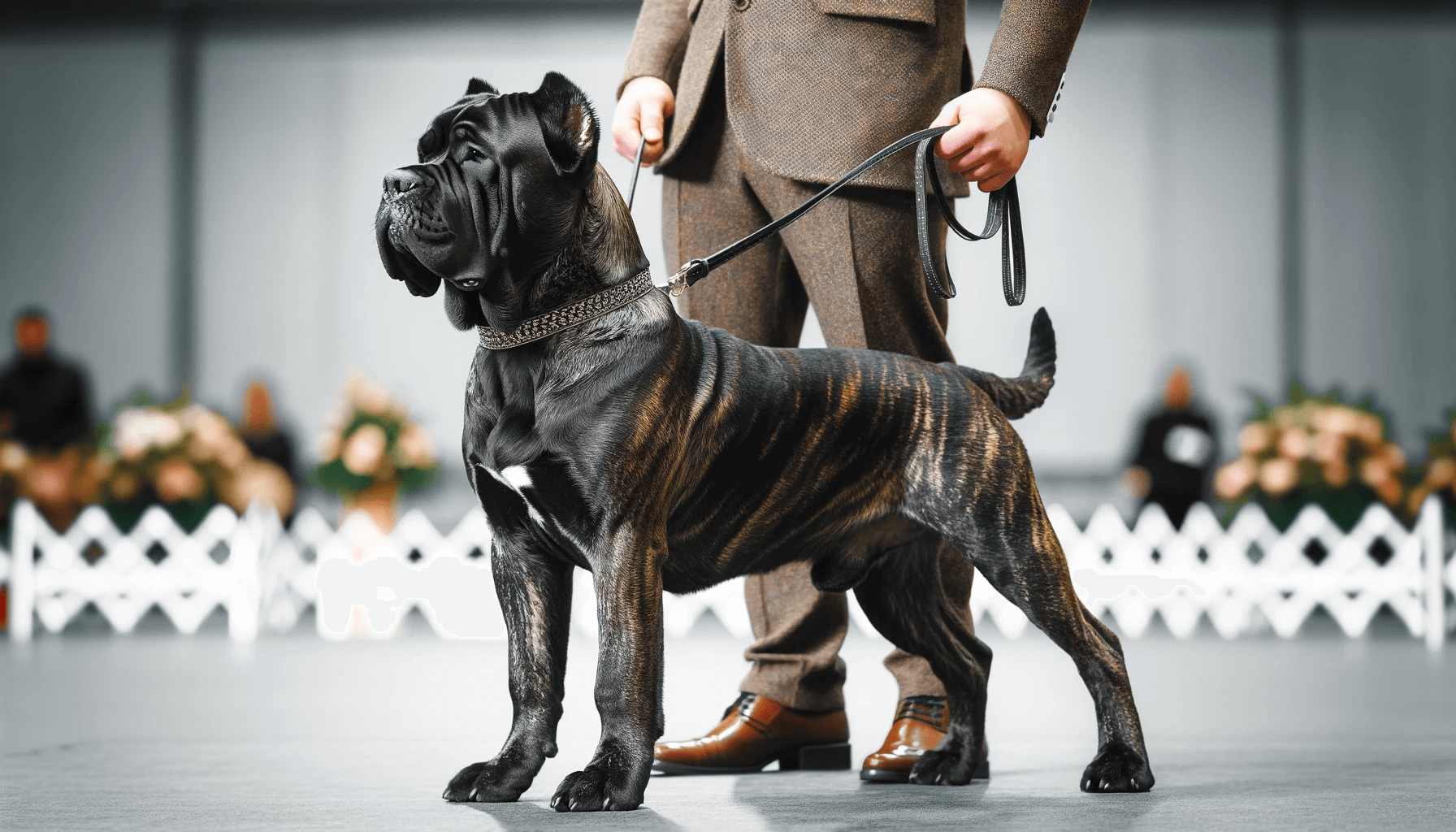In this detailed landscape-oriented color photograph, a Cane Corso is the primary subject, standing tall and alert in profile, with its gaze fixed to the left. The dog showcases a striking black coat with gold banding, a distinctive white Y-shaped marking on its chest, and a black muzzle adorned with jowly, wrinkled skin. The ears are small and pointed, adding to its noble appearance. Its stance is polished, with front paws firmly planted side by side and slightly spread back legs, while the tail curves gently upward. Likely at a dog show, the dog is held by its trainer, a man dressed in a brown tweed blazer, brown pants, and brown dress shoes, visible from the waist down. He grips a black collar and leash in both hands, securing the dog. The scene is set on a smooth, clean gray floor, with a slightly blurred, white picket fence in the background. Beyond the fence, blurry figures dressed in black and clusters of white, pink, and orange flowers complement the backdrop, enhancing the image’s representational realism style.